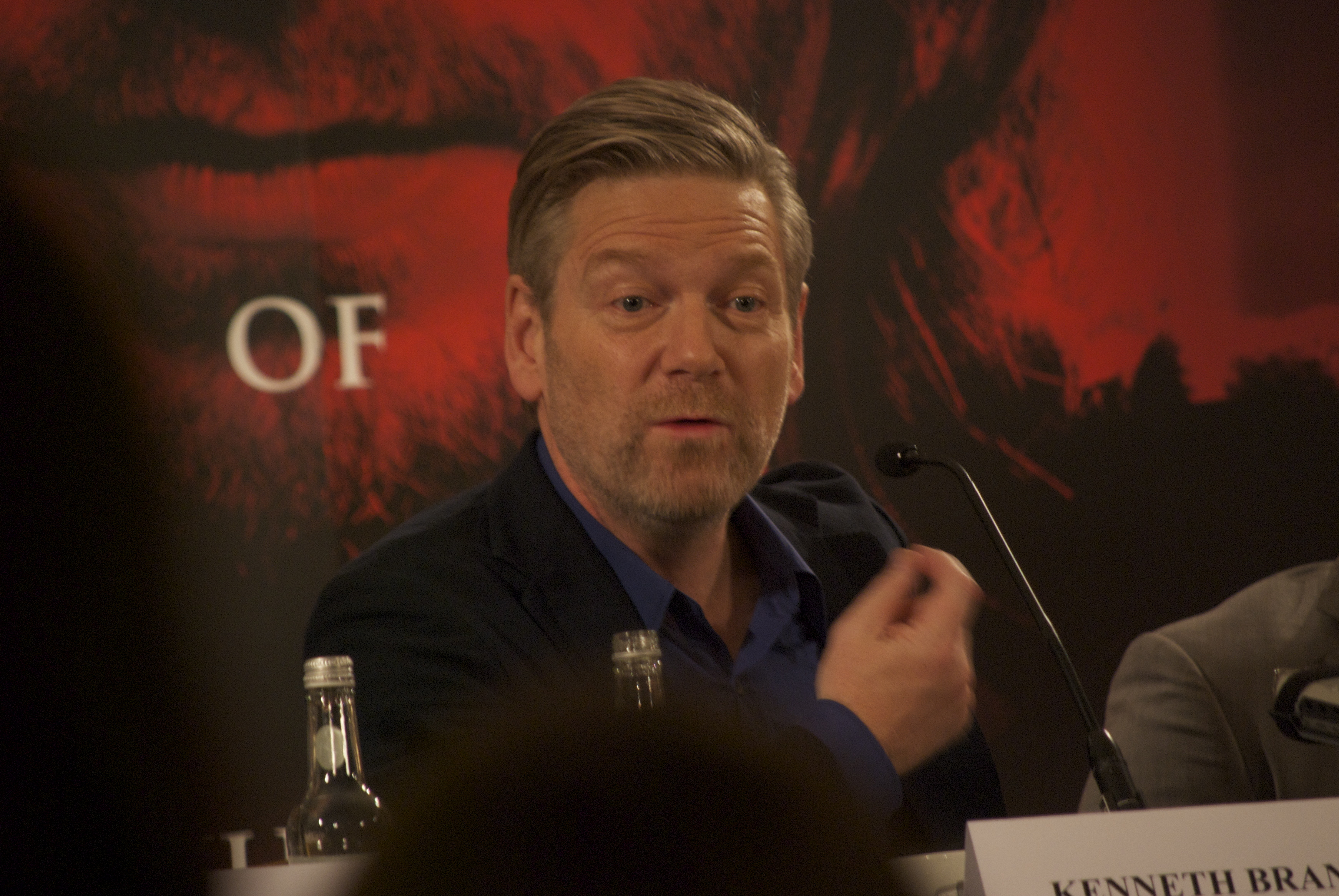The photograph features Director Kenneth Branagh seated at a table, possibly at a press conference. Branagh, a white male with blonde hair and a goatee, is mid-gesture with his right hand, suggesting he is speaking. He is dressed in a blue button-down shirt with an open collar, paired with a black blazer. In front of him lies a white paper nameplate that reads "Kenneth Branagh," though part of the sign is cut off. A small black microphone and two bottles, likely water, with silver caps are also positioned on the table. The background includes a partial blow-up image of what appears to be a movie poster, with the word "OF" being discernible.